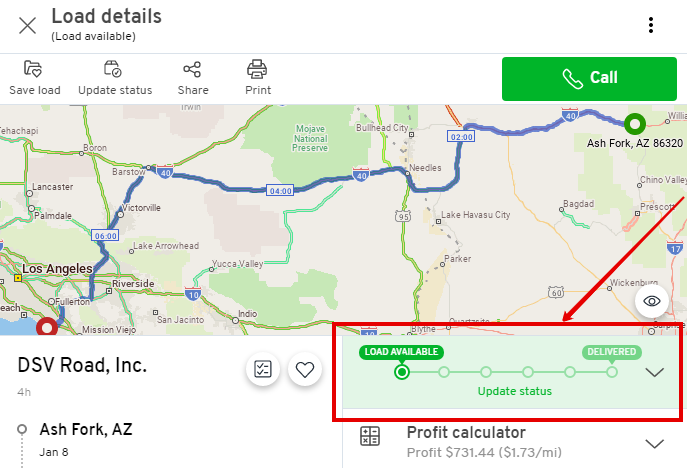The image displays a detailed logistics interface for a shipment route from Los Angeles, California to Ash Fork, Arizona, operated by DSV Road, Inc. The screen is encapsulated in a vibrant red box with a red arrow pointing towards several key interactive options, including 'Load Details,' 'Load Available,' 'Save Load,' 'Update Status,' 'Share,' 'Print,' and 'Call,' which is denoted by a green icon. Additionally, there are three dots in the top right corner, suggesting more options.

Central to the image is a map tracing the shipment’s route, marked with a zigzagging blue line that connects a red dot in Los Angeles to a green dot in Ash Fork. Along this route, various towns and key points are labeled, such as Ehupchoppe, Boron, Lancaster, Palmdale, Fullerton, Mission, Vallejo, Riverside, San Jacinto, Indio, Yucca Valley, Lake Arrowhead, Victorville, Barstow, Irwin, Mojave National Preserve, Bullhead City, Needles, Lake Havasu City, Parker, Blythe, Baghdad, Williams, Chino Valley, Prescott, and Wickenburg. 

Highways marked with blue shields bearing red tops, specifically Interstates 17 and 40, along with US Route 95, are shown tracing the path. Time estimates along the route indicate travel segments of 2, 4, and 6 hours. The surrounding geographic areas are color-coded with regions like the Mojave National Preserve highlighted in green and lighter green, while the rest of the map features a mix of gray and pinkish-brown hues. 

A profit calculator shows a profit of $731.44, translating to $1.73 per mile. Symbols for 'Print,' 'Share,' and a heart icon are also visible, adding to the interactive elements. This detailed interface provides comprehensive information necessary for logistics and route planning.